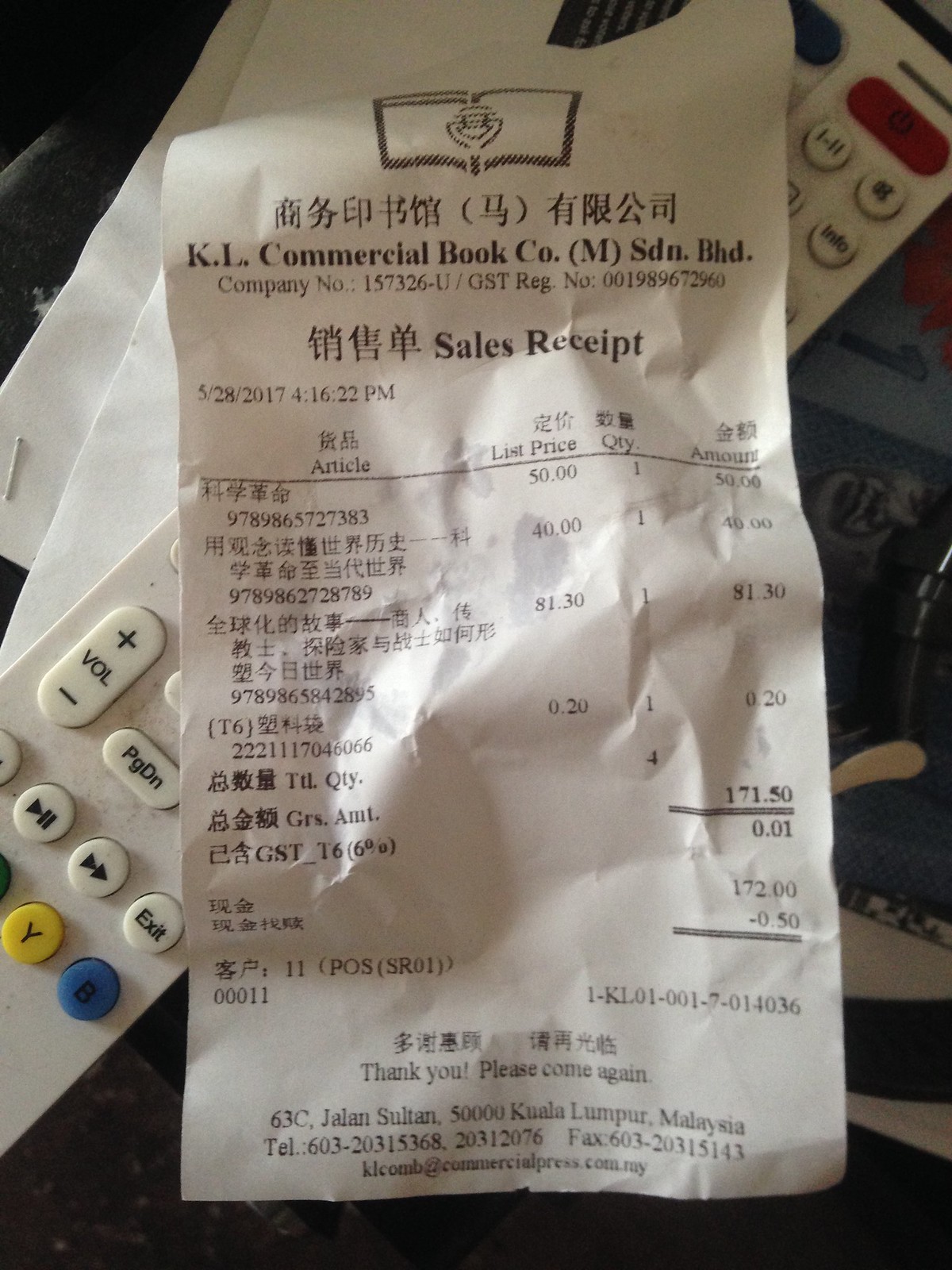**Detailed Descriptive Caption:**

The image features a color photograph displaying a wrinkled sales receipt placed on top of a television remote control. The remote sits on a sheet of white paper, secured with a visible staple in one corner. The remote control is predominantly white, adorned with round buttons in various colors: blue, yellow, and white, with a red power button positioned at the top. Each button is labeled with text. The receipt, originating from "KL Commercial Book Company," details the purchase of three books, with the titles written in an Asian language. The total amount on the receipt sums up to $171.50. It extends a courteous message at the bottom, reading "Thank you, please come again," followed by the company's address located in Malaysia. The overall color palette of the image features white and gray shades on the receipt, contrasted by the red, blue, and yellow buttons of the remote, adding vibrancy to the composition.